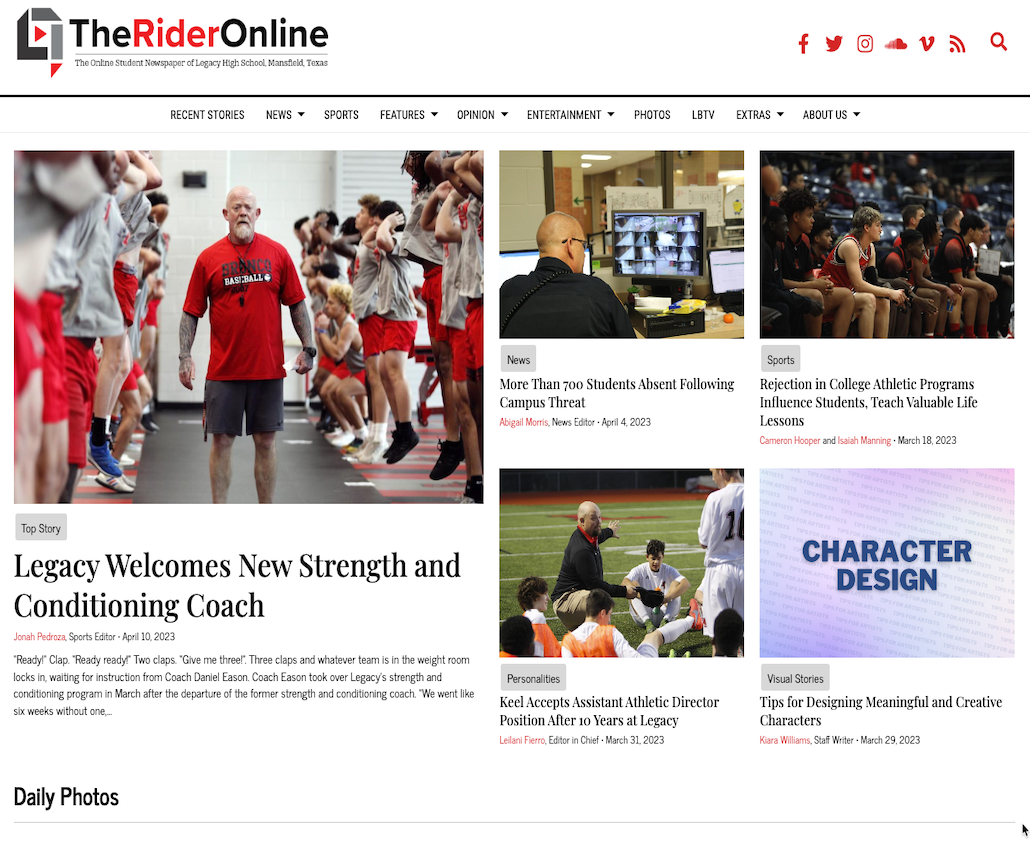This screenshot captures the homepage of The Rider Online, the student-run newspaper for Legacy High School in Mansfield, Texas. The layout features a clean, modern design with a prominent header containing navigation links. The main section displays several articles, each accompanied by vivid images. The top story highlights the school welcoming a new strength and conditioning coach, Daniel Eason. Other featured articles address various topics, including student absences following a campus threat, insights into college athletic programs, and tips for designing meaningful characters. The clear text sections and well-organized layout make for an engaging and accessible user experience.